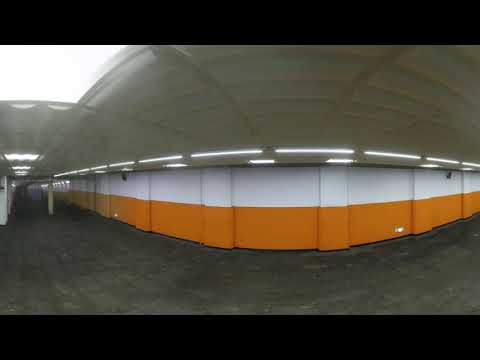This outdoor scene features a unique architectural structure that initially appears to be a parking lot but reveals itself to be more intricate. The building consists of a bottom section made of yellow bricks and an upper section of white bricks, topped with a gray dome adorned with interesting line patterns. At the base of the dome, there is a concrete area reminiscent of a sidewalk, extending backward where more dome-like buildings can be seen. The composition is mostly devoid of life or activity, with no vehicles or people present, creating an eerie and desolate atmosphere.

The wall displays a striking combination of colors and textures: an orange section that bulges in the middle and narrows at the ends, a white bar running across, and beige or gray arching structures with dark stripes. The foreground features a curved edge of dark gray concrete wrapping around the colorful wall. The scene is lit by the outside light evident in the cloudy sky visible in the upper left corner, suggesting overcast weather yet sufficient daylight illuminating the somber setting. The overall impression is of a stark, empty landscape with a sense of coldness and abandonment.